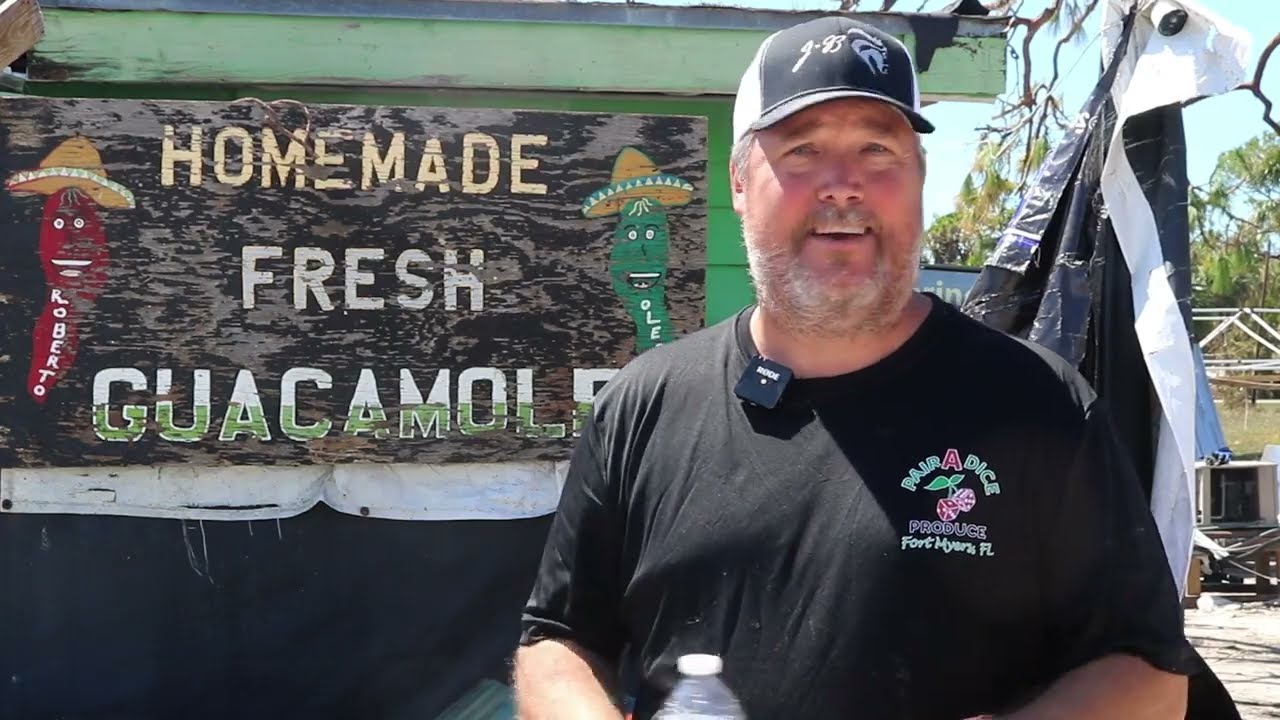In this vibrant outdoor photograph, a heavier-set Caucasian man with a round face stands front and center. His hair, beard, and mustache are a mix of white and dark brown tones. He is wearing a black and white baseball cap adorned with logos, including what appears to be a G, B, and a pelican. His mouth is slightly open, revealing some of his upper teeth. The man is dressed in a short-sleeved black t-shirt featuring the text "Paradise Produce, Fort Myers, Florida," with a distinctive design incorporating a pair of dice that resemble red cherries. A microphone is attached to his collar, and he holds a white water bottle in his right hand.

Behind him, a colorful sign proclaims "Homemade Fresh Guacamole," with the word "Homemade" in yellow text, "Fresh" in white, and "Guacamole" in white and green, against a backdrop that's half white and half green. Flanking the sign are two cartoon peppers wearing sombreros: a red one on the left labeled "Roberto" and a green one on the right with the partially readable text, "Ole". Further in the background, there's a green building and a clear blue sky with some trees, indicating a sunny day. A black and white flag is also visible to the right of the man.